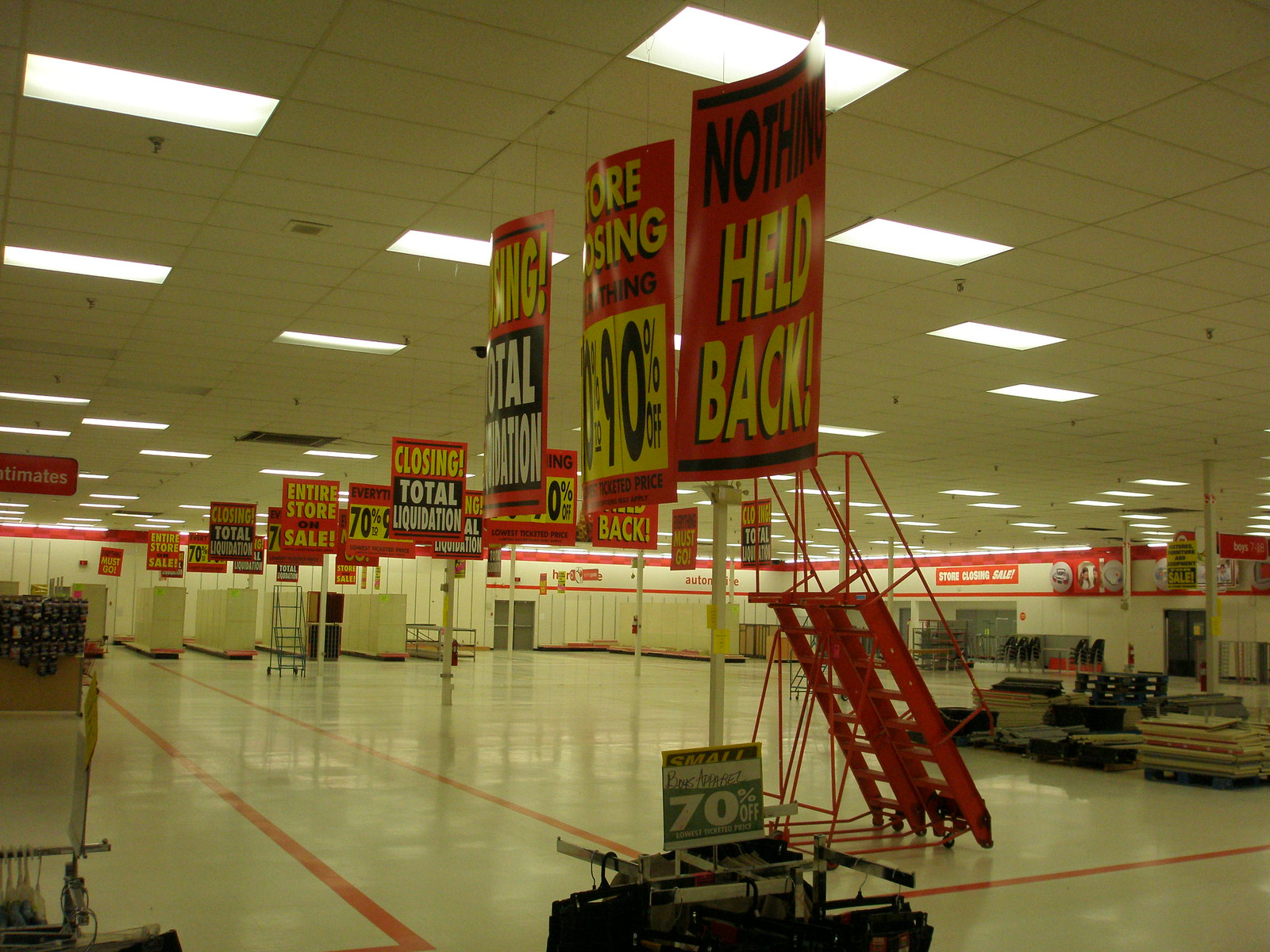The image depicts the interior of a large, deserted big-box store on the brink of closure. The scene features a vast, open space with a drop ceiling filled with rectangular fluorescent lights. White polished floors, marked with red lines delineating aisles and pathways, reflect the emptiness of the area. Most shelves have been removed, leaving a cavernous feel, and the remaining shelves stand barren. To the right, a stack of pallets is visible. Scattered signs declare the store's impending closure, announcing "Total Liquidation," "Entire Store Sale," and "Up to 90% off," amid other closing-related slogans. A few abandoned shopping carts sporadically dot the space, and a red rolling ladder with handrails, positioned near a post bearing some of the signs, adds to the atmosphere of finality and vacuity.